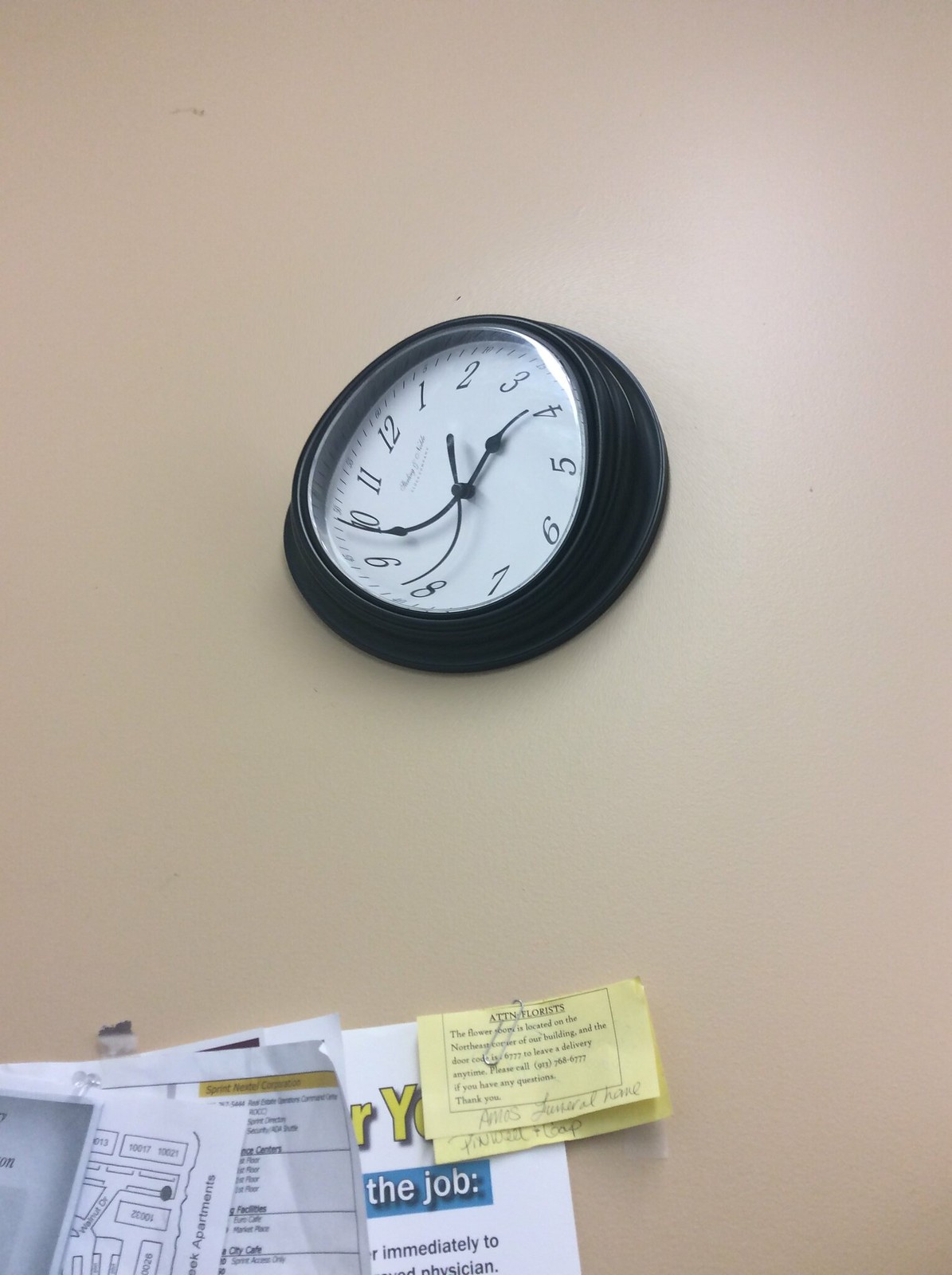In this image, a clock prominently hangs on a cream-colored wall. The clock features a traditional design with a black frame, a white face, and black hands. Interestingly, the clock appears to be unnaturally skewed, as if viewed through a fisheye lens, giving it a distorted and sideways look. However, the alignment of several papers neatly thumbtacked or taped below the clock indicates that this distortion is likely intentional in the clock's design, as the papers themselves remain perfectly straight and unaffected. The contrast between the clock's warped appearance and the orderly papers beneath it adds a curious and intriguing visual element to the scene.